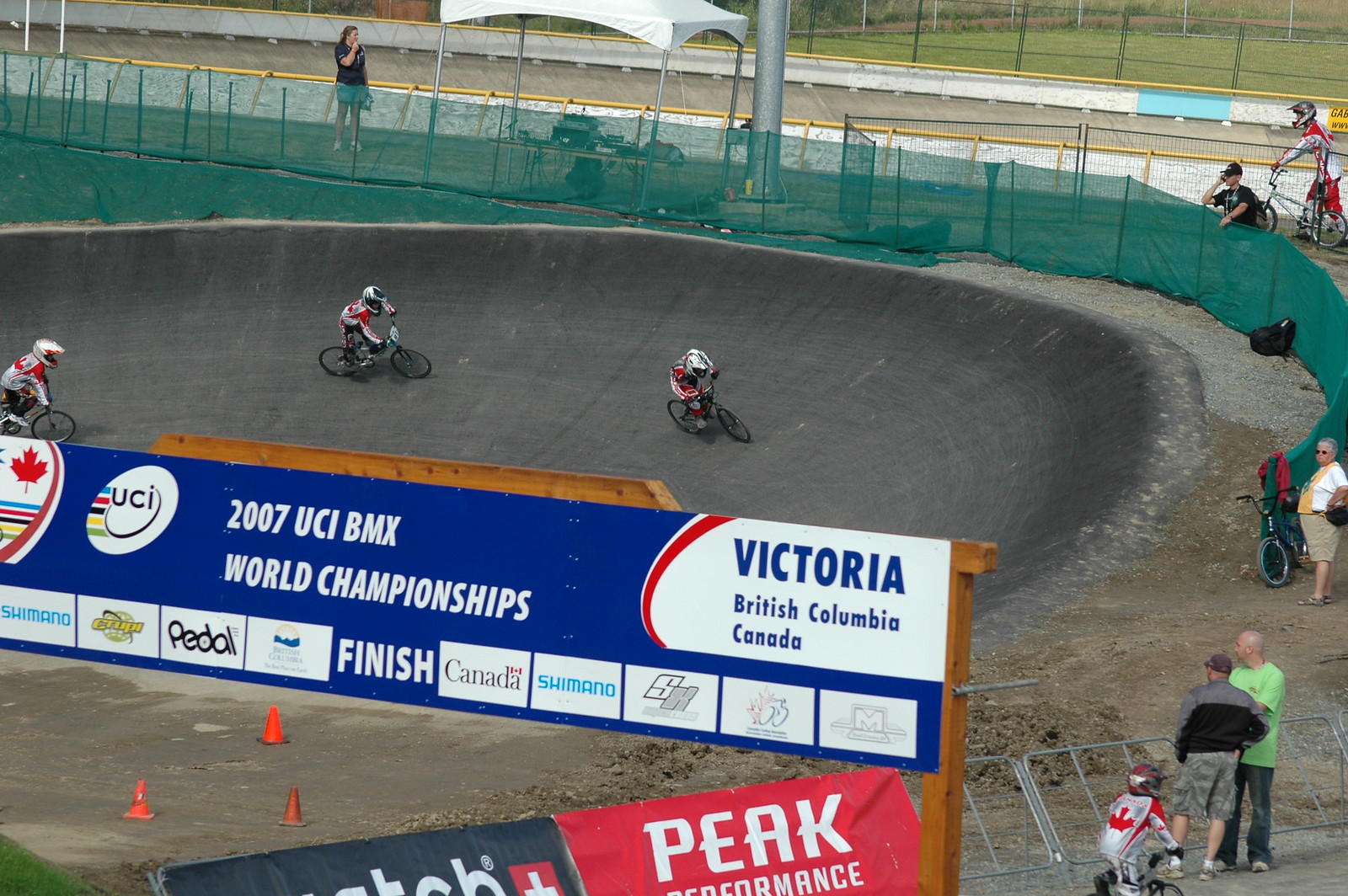The image depicts the 2007 UCI BMX World Championships in Victoria, British Columbia, Canada. Three riders, sporting white helmets and red jerseys, are racing on a dark gray, dirt BMX track that curves upward around a corner. A large blue banner is prominently displayed in the foreground, secured on wooden poles, and reads 'UCI BMX World Championships' with 'Victoria, British Columbia, Canada' written at the bottom in white squares, featuring the names of various sponsors like Shimano and Peak Performance. The track is surrounded by green fencing, with spectators observing the race from an elevated platform area above the track. Additionally, some orange cones are present, adding to the competitive atmosphere, while patches of grass can be seen in the background.